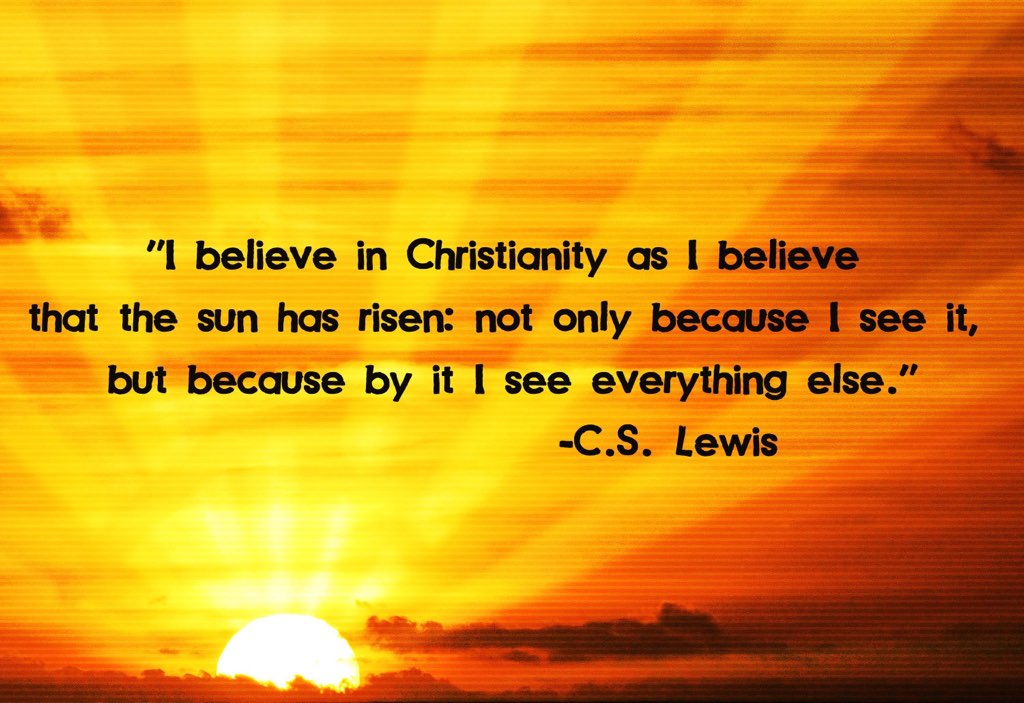A captivating image features a bold black C.S. Lewis quote set against a stunning sunrise. The quote reads, "I believe in Christianity as I believe that the sun has risen, not only because I see it, but because by it I see everything else." The background is a picturesque sunrise with vibrant hues of yellow, orange, and red that paint the sky, creating a striking contrast with the text. Six distinct beams of yellow light radiate across the sky, with half of the glowing sun either behind a cloud or ascending from behind a mountain, adding depth and drama to the scene. This visually appealing combination of the quote and the sunrise backdrop makes for an inspiring and shareable image that could easily be printed or posted online.